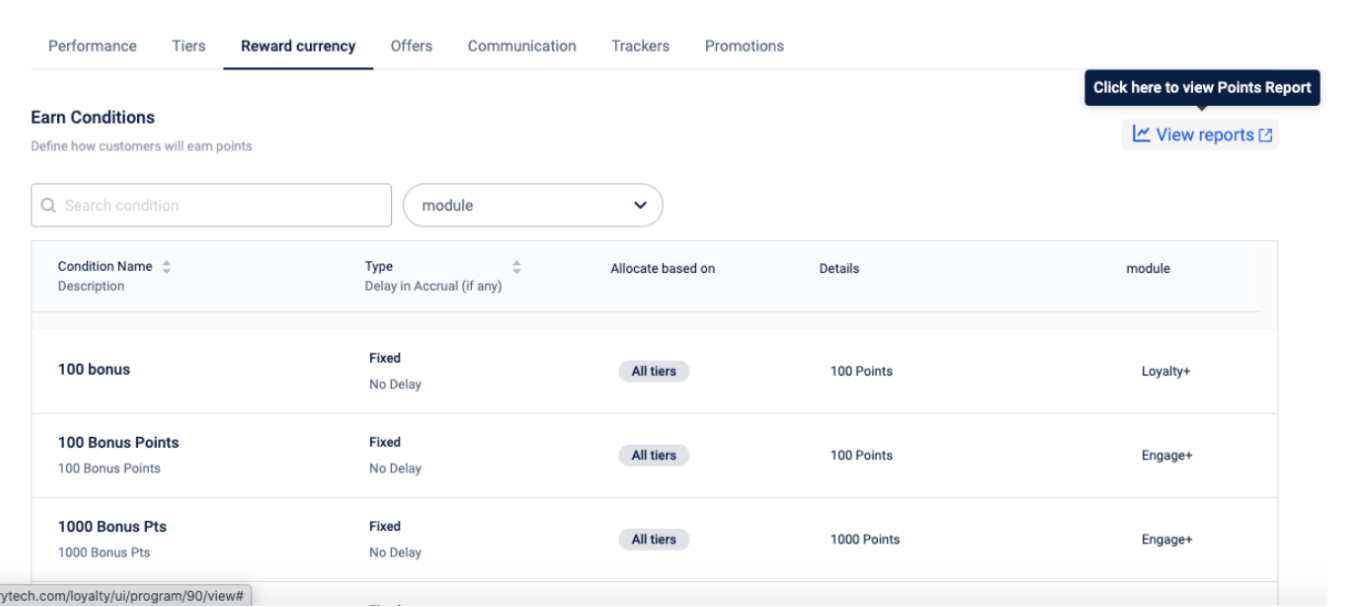The screenshot displays a comprehensive overview of the Reward Currency section within a user interface. Along the top, several navigational tabs are visible: Performance, Tiers, Reward Currency, Offers, Communication, Trackers, and Promotion. The Reward Currency tab is currently active, displaying the Earn Conditions section. Just below, there is a search box accompanied by a drop-down menu labeled "Module."

The main content of the screenshot features a list of four rectangular entries organized in a grid format with columns labeled as follows: Condition Name, Type, Delay and Approval, Allocate Based On, Details, and Module. 

- The first rectangle in the list displays:
  - Condition Name: "100 Bonus"
  - Type: "Fixed"
  - Delay and Approval: "No Delay"
  - Allocate Based On: "All Tiers"
  - Details: "100 Points"
  - Module: "Loyalty Plus"

- The second rectangle mirrors the first with slight variations:
  - Condition Name: "100 Bonus"
  - Type: "Fixed"
  - Delay and Approval: "No Delay"
  - Allocate Based On: "All Tiers"
  - Details: "100 Points"
  - Module: "Engage Plus"

- The third rectangle down similarly displays:
  - Condition Name: "1,000 Bonus"
  - Type: "Fixed"
  - Delay and Approval: "No Delay"
  - Allocate Based On: "All Tiers"
  - Details: "1,000 Points"
  - Module: "Engage Plus"

In the top right-hand corner of the screenshot, a "View Reports" button is prominently placed, alongside a notation that instructs users to "Click Here to View Points Report." This setup provides a clear, concise summary of the different reward conditions, types, and associated details for each module, facilitating the management of reward currencies within the system.